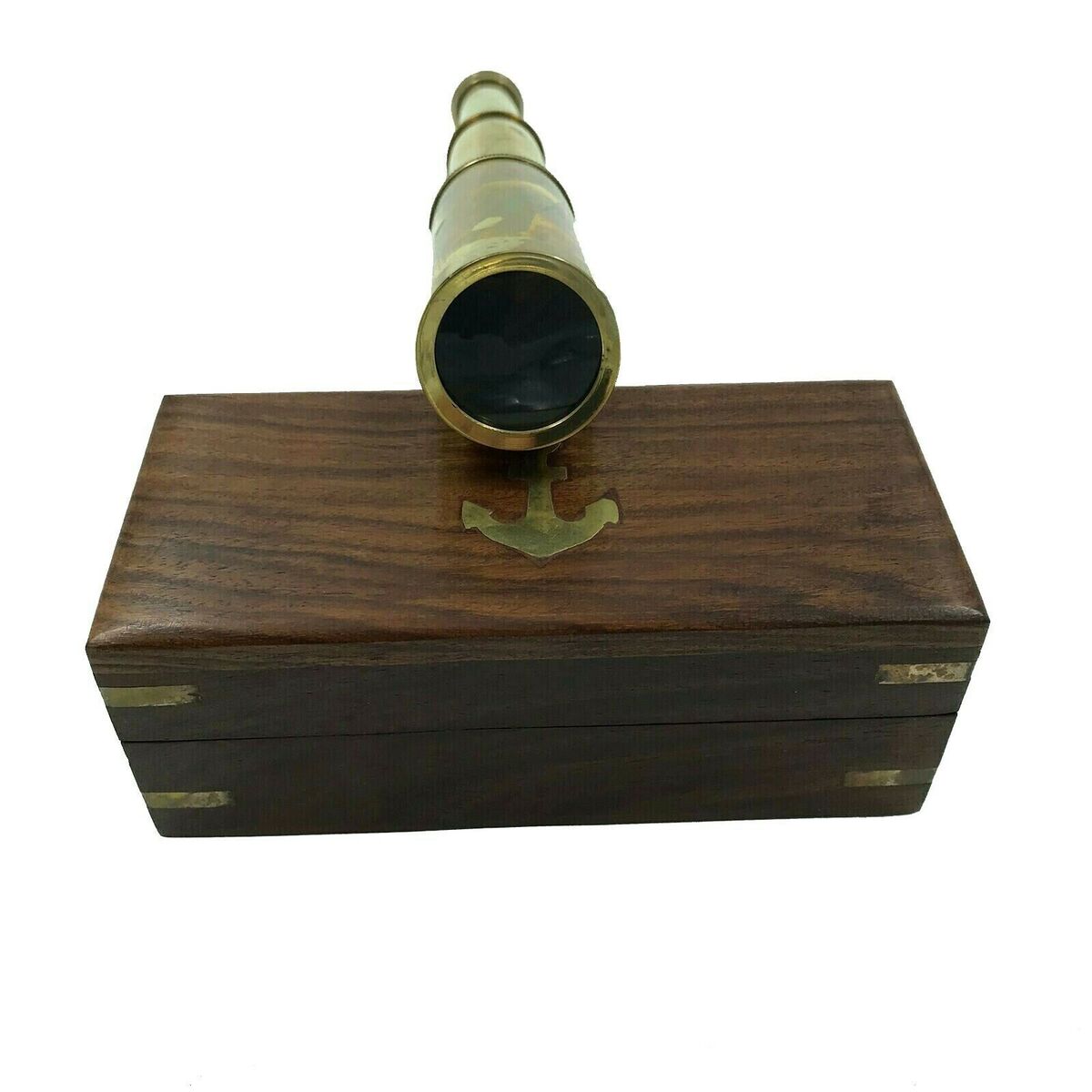The image depicts a detailed product photo set against a plain white background, showcasing an antique-style wooden box with brass inlays on its corners and a decorative brass anchor on its top. The box, crafted from dark brown wood with a simple, aged finish, features slightly oxidized brass fittings, giving it a vintage appearance. Resting upon the box is an old-fashioned brass telescope, reminiscent of those used by sea captains or pirates during the 1800s. The telescope, with its brass construction and patina finish from apparent aging, is extended in three sections and positioned to display the open end, enhancing its authentic vintage charm.